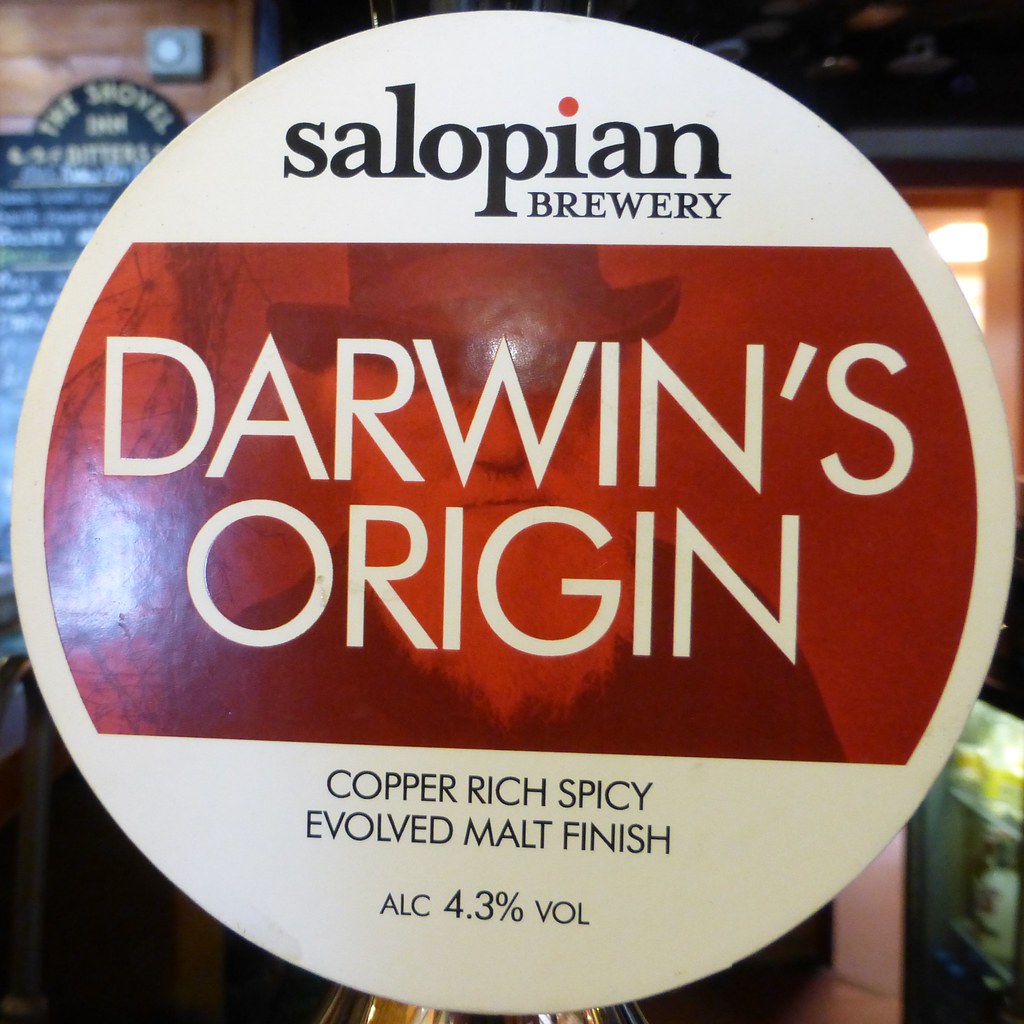The image is a square photograph taken inside a pub or restaurant with a warm, inviting atmosphere highlighted by wooden paneling and an out-of-focus chalkboard listing in the background. The focal point is a circular sign attached to the top of a beer tap, with a glimpse of the brass tap visible below. The sign features a white background and prominently displays "Silopian Brewery" in black text at the top, with the red dot in the letter 'i'. Beneath that is a red stripe area featuring a vintage black-and-white image of a gentleman with a bushy white beard and a top hat, resembling Charles Darwin, tinted in red. Overlaid on this red area in white text is "Darwin's Origin", followed by a description underneath on the white background, in black text, that reads "Copper-Rich Spicy Evolved Malt Finish, ALC 4.3% volume". The photograph also captures a hint of the bar area to the left, with a dark area possibly indicating the bar counter, and a refrigerator visible in the lower right.